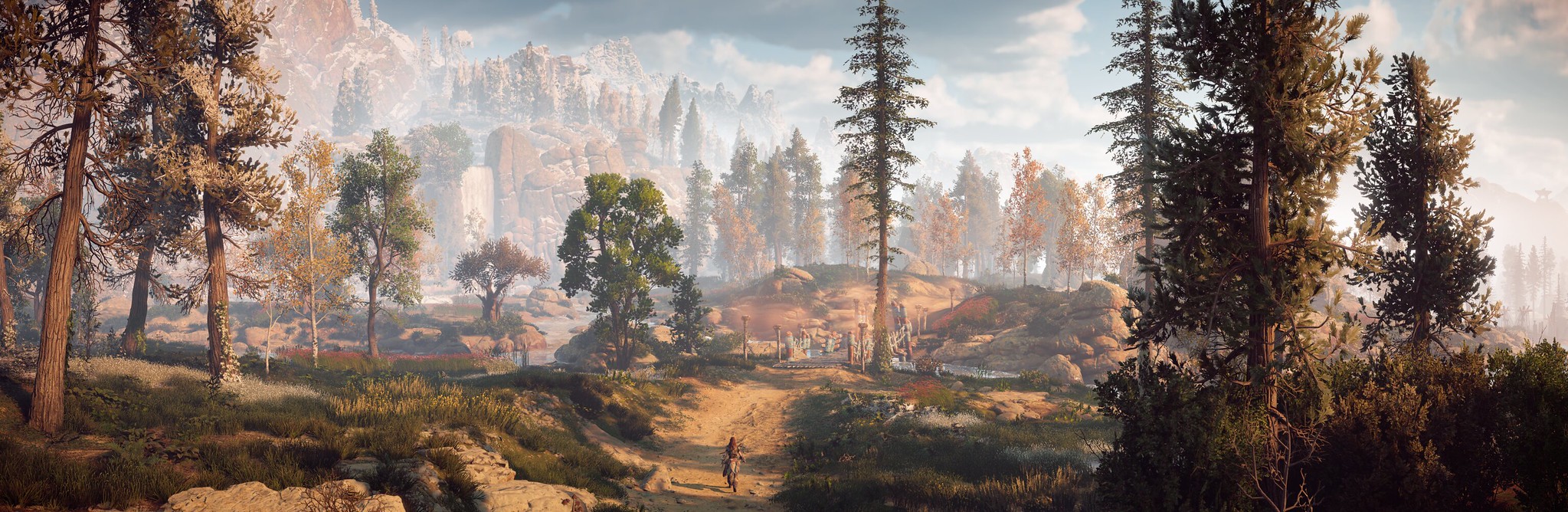This image captures a breathtaking scene from a video game, depicting a vibrant and lush forest landscape. The forest is a mosaic of green, red, and yellow foliage, showcasing nature in its full glory. A winding road meanders from the bottom center of the image, extending towards the distant horizon, inviting exploration. Dominating the background, a majestic mountain range is crowned by a stunning waterfall cascading down its slopes, adding a dynamic and serene touch to this virtual wilderness.